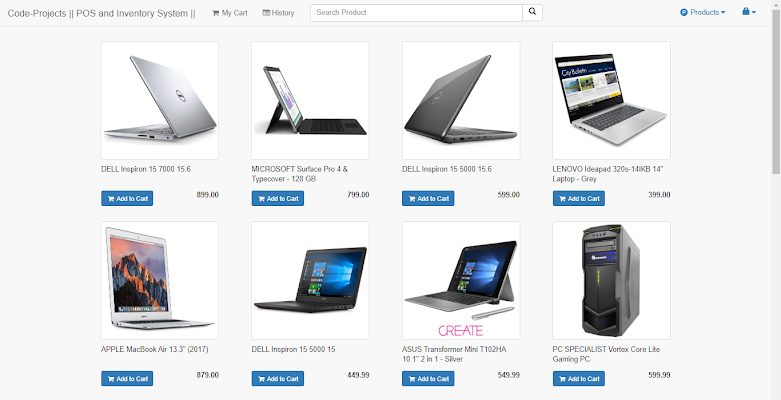The screenshot depicts a shopping webpage titled "Code Projects POS Inventory System." In the top-left corner, options include "My Cart" and "History," alongside a search bar labeled "Search Products." On the right, there is a section named "Products" featuring images of padlocks.

Below this section is a list of selectable products, each featuring an image, product description, an "Add to Cart" button, and prices, although the currency is not specified. The products listed are primarily laptops and one desktop computer:

1. **Dell Inspiron 15 7000**, 15.6-inch, priced at $899
2. **Microsoft Surface Pro 4 with Type Cover**, 128GB, priced at $799
3. **Dell Inspiron 15 5000**, 15.6-inch, priced at $599
4. **Lenovo IdeaPad 320S**, 14KB, 14-inch, gray, priced at $399
5. **Apple MacBook Air**, 13.3-inch, 2017 model, priced at $879
6. **Dell Inspiron 15 5000**, 15-inch, priced at $449.99
7. **Asus Transformer Mini T120HA**, 10.1-inch, silver, priced at $549
8. **PC Specialist Vortex Core Lite Gaming PC**, a computer tower, priced at $599.99

Each product has a clear image, detailed description, and dedicated "Add to Cart" button for easy shopping functionality.